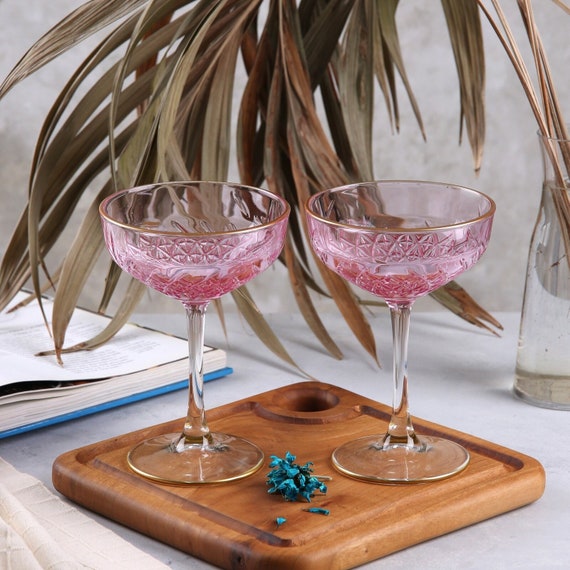The photograph captures a sophisticated indoor setting featuring a white tabletop on which a light brown, wooden square cutting board is centrally positioned. Atop this cutting board are two empty, pink margarita glasses with gold rims and clear stems. Scattered between these glasses are delicate blue petals, resembling dried flowers. To the left of the cutting board, an open book partially intrudes into the frame, along with a white tablecloth peeking into the scene. Beyond the cutting board to the right, a tall, translucent glass vase filled with water stands, showcasing a dramatic arrangement of olive-colored, palm-like fronds with brown stems that arc gracefully over the setting. The overall composition exudes an air of casual elegance with a rustic touch.